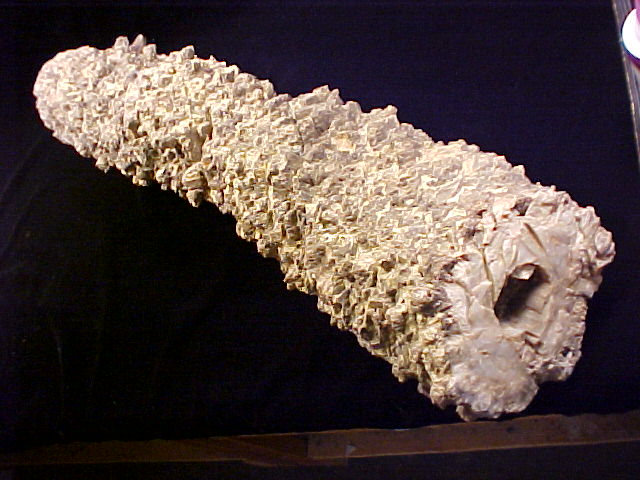The image depicts what appears to be an ancient, cylindrical artifact with a cream-colored, rough surface adorned with numerous extensions and a central hole. The artifact, resembling a naturally occurring rock or coral structure, features a long, rocky, and rigid appearance that could suggest geological origins. It is housed in a museum exhibit, placed within a purple-colored container. The background of the exhibit includes a black sheet or cloth, with a top right area showing hints of white, red, and silver elements. At the base of the container, there is a brown wooden plank that encircles the artifact. The overall shape of the image is rectangular.